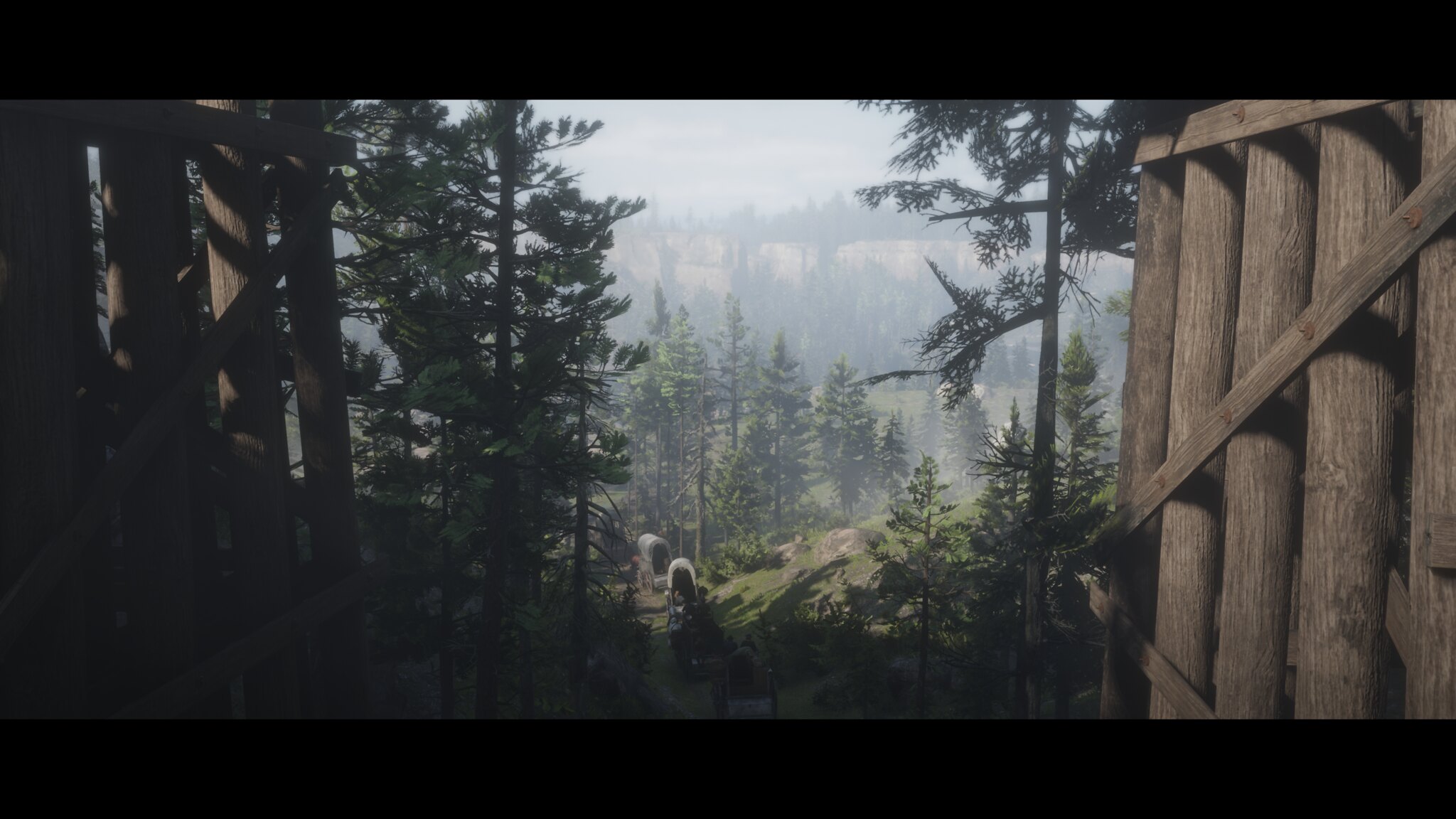This screenshot from a video game presents a vivid, cinematic view as if the viewer is standing behind a set of opened wooden gates. These gates, which possibly feature angled wooden planks, frame a grand wilderness setting characterized by an expansive valley filled with a dense array of tall, green trees, including pine trees. The valley stretches far into the distance, becoming increasingly hazy and cloud-like as it disappears into the horizon, adding to the sense of vastness. The sky above reflects this haze, casting a soft, ethereal light over the landscape. In the foreground, a defined trail meanders up towards the gates from within the valley. On this path, covered wagons drawn by horses make their way uphill, contributing to the scene's immersive and detailed environment. The overall image is surrounded by a flat, jet-black background, enhancing the focus on the central, richly detailed outdoor scenery and its encompassing wilderness.